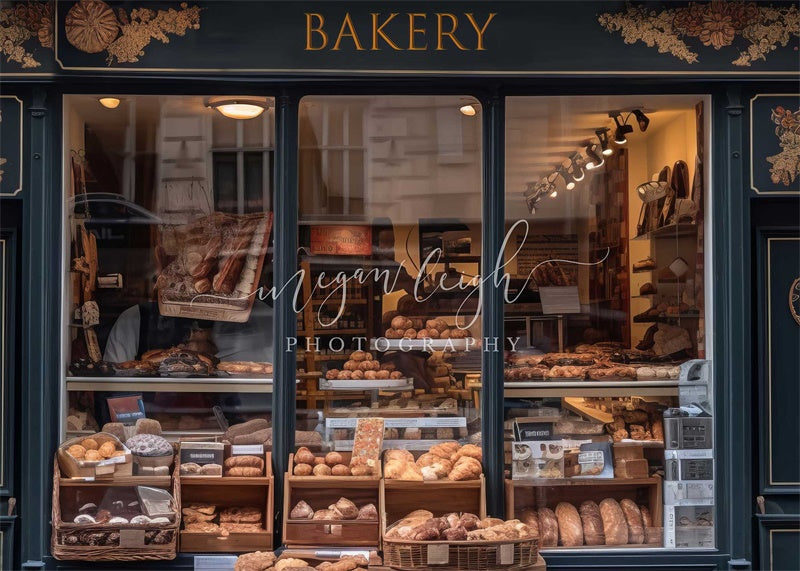The image depicts a charming storefront of a deep blue-colored bakery adorned with intricate gold floral designs. Prominently displayed above the entrance is the word "BAKERY" in capital letters, etched in gold. The bakery's front features three long glass windows, allowing a clear view of the inviting interior. Reflected in the glass are the cream-colored brick buildings across the street. Superimposed on the window is the text "Megan Leigh Photography," indicating the photographer. Inside, an array of golden brown breads, rolls, pastries, and baguettes are meticulously arranged in baskets and trays. A person, possibly a customer or an employee, can be seen in the background amidst the warm ambient lighting, adding a touch of lively activity to the cozy scene.